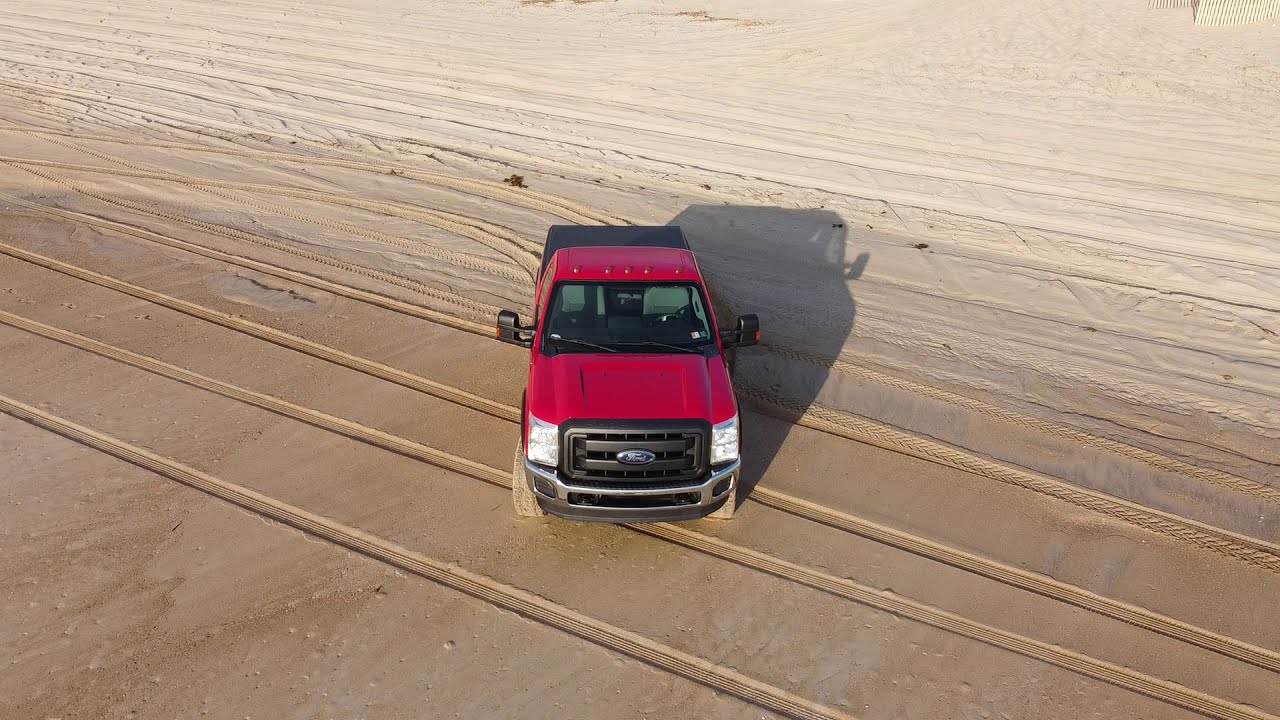In this detailed aerial image, we see a ruby red Ford 4x4 pickup truck, facing towards the camera. The truck exhibits distinctive features such as a prominent front black grille with the iconic blue Ford oval logo, stacked headlights, and black side-view mirrors. The windshield appears slightly tinted, revealing two whitish bucket seats within the black interior, although there's nobody inside. The truck bed is covered with a black cover and adorned with exterior marker lights on the roof. The pickup is stationary on a sandy surface marked by parallel lines and crisscrossing tire tracks, indicating previous movements, possibly from off-roading activities. The sand transitions in color from a wet, reddish-brown near the truck to a drier, beige hue in the distance, creating a pattern suggestive of varying moisture levels, possibly from recent wave activity. The sandy terrain reveals a mixture of wet and dry textures, adding depth and complexity to the scene.